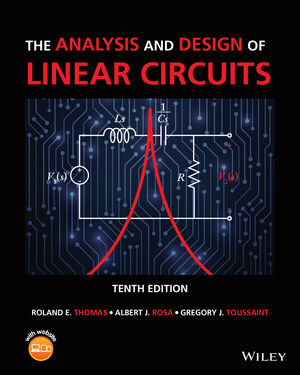This image is the cover of a book titled "The Analysis and Design of Linear Circuits," prominently featuring its title in red font for major words and white font for minor words, set against a black background. At the center of the cover is an image depicting an electrical diagram of a circuit, complemented by a mirrored red curved line on both sides. Below this central image, the text "10th Edition" is displayed in white font. Underneath, the names of the authors—Roland E. Thomas, Albert J. Rosa, and Gregory J. Toussaint—are listed in alternating red and white font. In the bottom right corner, the publisher's name, Wiley, is clearly visible, while the bottom left corner features an orange circle logo, presumably associated with the textbook company.